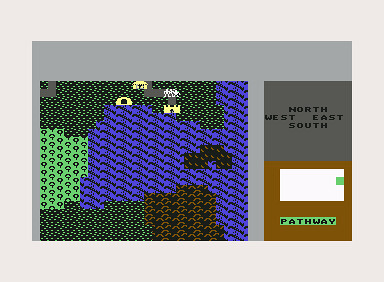The image appears to be a screenshot from a video game featuring a detailed map. The right-hand side of the map shows a gray square. Labels indicating North and South are present, with North on the left and South on the right. Below these labels, the landscape transitions through several colors: brown, white, and multiple shades of green, leading into what appears to be a green pathway bordered by black sections.

At the top of the map, there is a densely green area with lighter green dots, suggesting vegetation or trees. Nestled within this greenery is a distinct yellow cave with a black entrance. Scattered across the map, gray roads intersect various buildings.

On the left side of the map, there is a light green field dotted with trees, while on the right side, a lake is depicted with blue water and surrounding stone formations. The bottom of the map features a grid of black squares with brown centers, interspersed with numerous small dots, hinting at a complex, perhaps inhabited area.